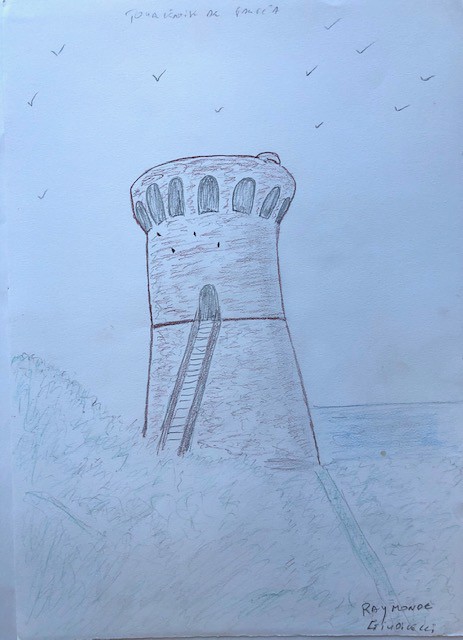This is a detailed pencil drawing rendered on light blue paper, depicting a solitary cylindrical tower atop a high, grassy hill. The tower is characterized by its slightly wider lip at the top, which features a series of arched windows encircling its upper section. A narrow stairway ascends from the base of the hill to an arched wooden door that serves as the tower's entrance. In the background, a vast body of water—possibly a large lake or the ocean—stretches out, complementing the serene scene. Birds are depicted soaring overhead, adding a sense of movement and life to the tranquil setting. A winding trail meanders up the hill from the base, leading directly to the tower. The artist's name is signed in the bottom right corner of the drawing.